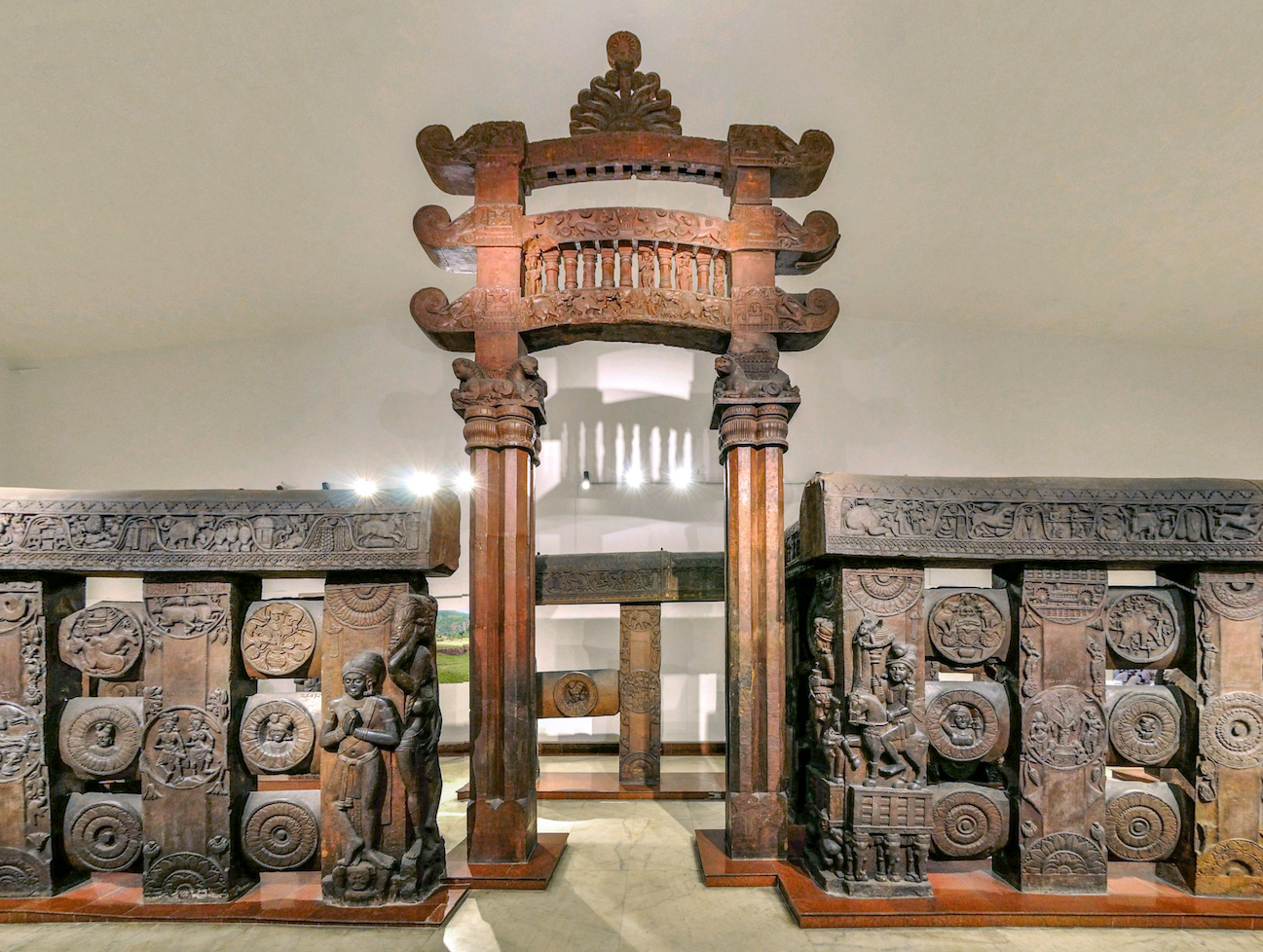The image depicts a highly detailed, scale model of a traditional Chinese architectural gateway, constructed from wood. Central to the composition is the ornate arch-shaped entrance, which features a honey-colored wooden gate flanked by two robust wooden columns, connected at the top. Above the arch, intricate curlicue designs extend outward, culminating in a crown-like shape adorned with floral carvings resembling a pineapple's leaves.

On either side of the main archway, there are elaborate stone walls and rectangular wooden panels, each meticulously decorated with carvings of human figures, animals, and circular medallions with detailed engravings. The wooden structures of the walls display a variety of hues, from honey-colored to grayish brown, highlighting the intricate craftsmanship. The entire setup, resembling a one-story tall building, is likely housed within a museum or gallery, showcasing the traditional and artistic essence of ancient Chinese architecture.